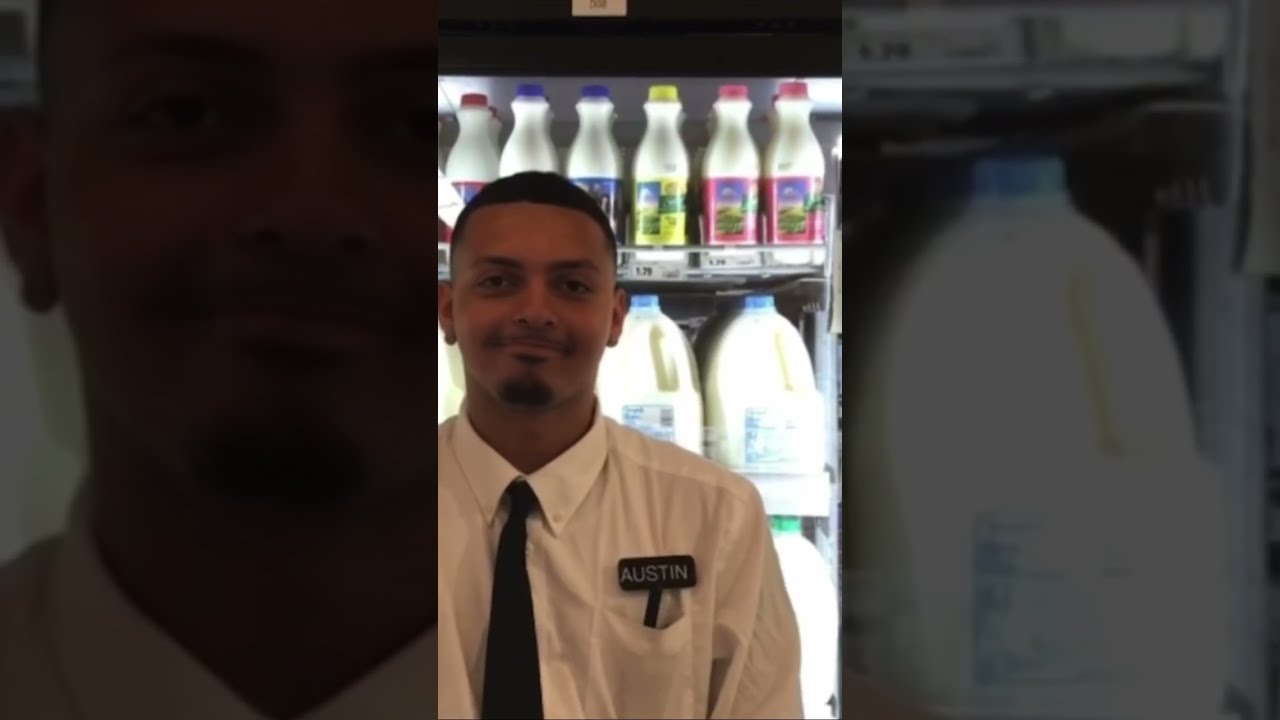This graphic depicts a prominently featured portrait of a young man of African descent with light brown skin, dark black hair, a small goatee, and a mustache. He appears to be possibly wearing earrings, and he is dressed in a white button-down long-sleeved shirt with a black or dark tie. A black rectangular name tag with white letters reads "Austin" above his pocket, where he also keeps a pen or pencil. The man is smiling slightly, suggesting a friendly demeanor, and stands in front of a refrigerated display filled with gallon to pint containers of milk. This central portrait is vertically oriented and occupies the middle section of the wide, landscape-oriented graphic.

On either side of the central image, the graphic is divided into two darker, close-up panels. The left panel provides a zoomed-in, shadowed view of Austin's smiling face, emphasizing his expression. The right panel offers a similar close-up, darkened view of a gallon of milk from the display behind him. This careful arrangement highlights Austin in the center, drawing attention to his role in what appears to be a grocery store or gas station setting, likely as an employee overseeing the milk section.